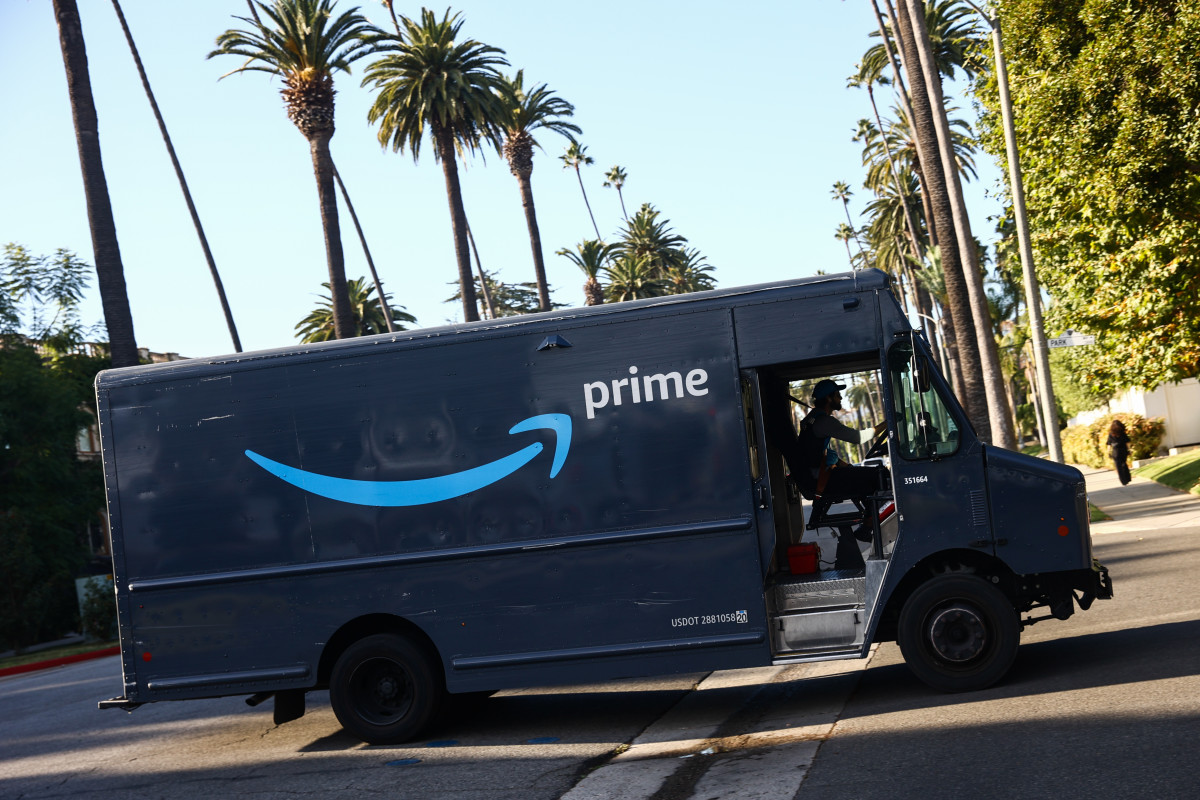In this vibrant image, a dark blue Amazon Prime van is prominently featured. The vehicle is positioned slightly higher on the right side due to the angled roadway, with its front end facing left and its rear to the right. Notably adorned with the distinctive Amazon arrow logo and the word "Prime" just before the side door, the van also sports black wheels and rims. The side door is open, revealing the silver flooring inside and a solitary black chair.

The setting around the van is detailed with various natural elements. Directly in front of the step-up into the van, the road slightly inclines, with two white lines stretching underneath the vehicle. Green bushes are visible to the left of the van, while a line of trees stretches across its background. These include a mix of shorter trees and taller palm trees.

In the foreground, a woman dressed entirely in black walks along a gray sidewalk. Bushes and a white fence line her path, and a towering green tree extends upwards, partially covering the scene. The sky above is a clear, striking blue, providing a serene backdrop to the bustling environment below.